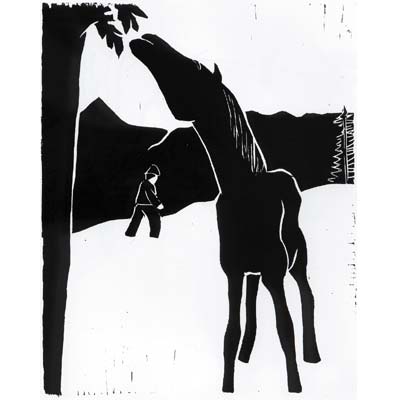This black and white illustration, "Horse Feeding from a Tree" by Werner Berg, created in 1933, is a woodcut in the expressionist style. In the center of the image is an all-black horse with a long neck extended towards the upper left, reaching for leaves or possibly an apple from a tree. The tree's trunk runs along the left edge, with leaves hanging down toward the horse's face. The horse's legs are elongated and cut off at the bottom, adding to its shadowy, almost abstract appearance. A small figure of a man dressed in black occupies the center-left background, walking towards the right. Behind the man, simplistic mountains and hills shape the background. Black markings in the upper right and bottom left corners contribute to the minimalist yet striking contrast against the white, signifying a clear sky. The entire composition is rendered with black, white, and shades of gray, highlighting the artwork's expressionist nature and emphasizing the stark contrast and emotional depth.